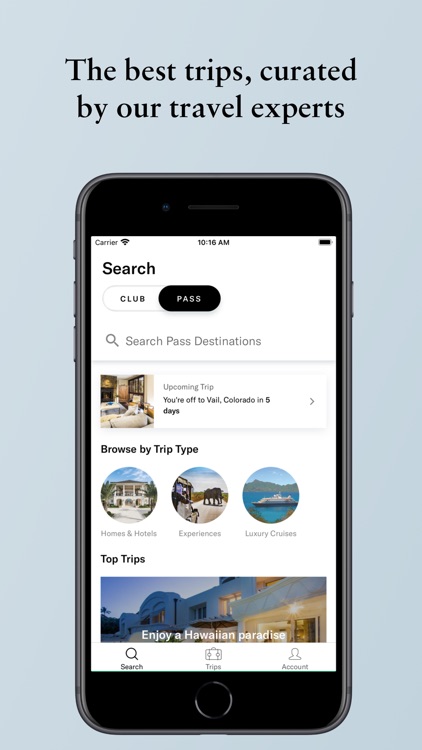A vertical photograph features a sleek cell phone set against a gray-blue background. At the top of the image, in bold black lettering, reads the heading: "The Best Trips, curated by our travel experts." Directly beneath the heading is the outlined silhouette of the cell phone, which has a dark gray or black housing with black sections at both the top and bottom.

The phone’s screen displays detailed information. In the top-left corner, it shows the label “Carrier” and a Wi-Fi icon, while the center of the screen displays the time "10:16 AM." On the top-right corner, there’s an almost fully charged battery icon.

Scrolling down, on the left-hand side in bold lettering, the word “Search” appears next to a toggle button. The toggle button has two sides: on the left, it’s white and marked “Club,” while on the right, it’s black and marked “Pass.” Below this, on the left side, there's a search magnifying glass icon labeled “Search Past Destinations."

In the middle of the screen, there is a small photograph of a cozy, inviting living room labeled “Upcoming Trip.” Accompanying this image is a message indicating that the next destination is Vail, Colorado, in five days, followed by a right arrow suggesting further details.

Further down, the section labeled "Browse by Trip Type" showcases three circular icons. The first icon displays a mansion-style building under the label “Homes and Hotels.” The center icon features a Jeep on a dirt road with an elephant crossing, labeled “Experiences.” Lastly, the third icon shows an ocean with mountains in the background and a cruise ship in the middle, labeled “Luxury Cruises.”

The final section of the screen is titled "Top Trips." Here, a horizontal rectangular image illustrates the caption "Enjoy a Hawaiian Paradise," featuring a lit-up white building.

At the bottom of the screen, navigation options are displayed: "Search" on the bottom left, "Trips" in the center, and "Account" on the far right.